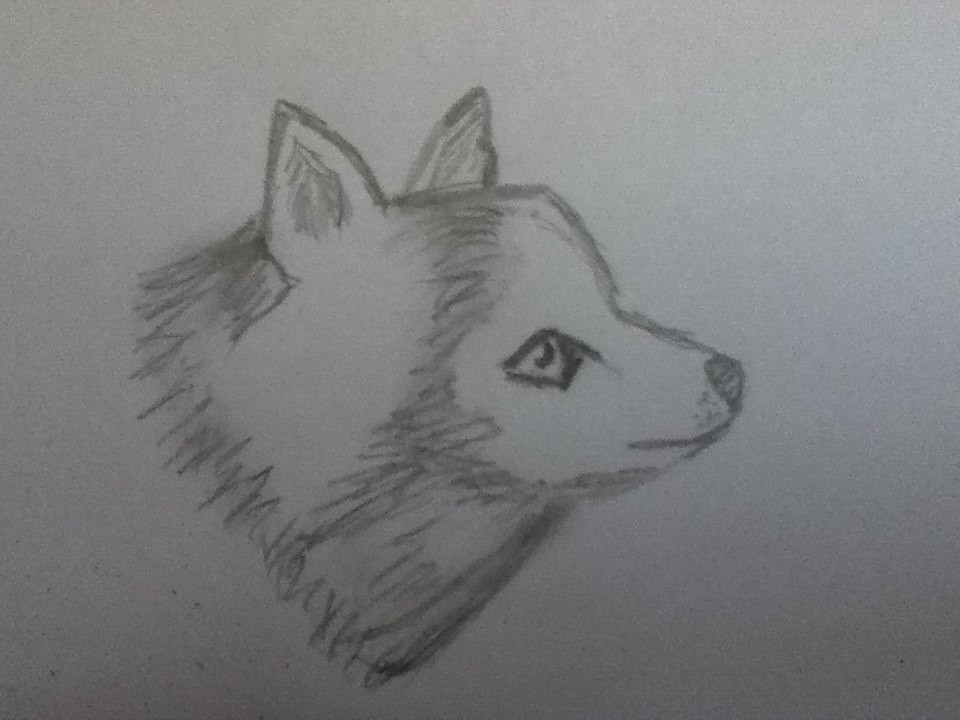The image features a side profile drawing of a canine-like animal, possibly a fox, dog, or wolf, rendered in pencil on white paper. Centered on the page but not filling it entirely, the drawing captures the head and a small portion of the neck. The creature has two upright, pointy ears and a distinctly dark, thickly outlined eye with a small highlight, contributing to a somewhat human-like appearance. The shading around the eye, ears, and nose, as well as beneath the ears, is simplistic but provides necessary definition. The nose is gray and the mouth is delineated by a simple line with small dots below to indicate whiskers. Despite its crude and basic style, the drawing features fine pencil lines to suggest fur, showing a modest range of shading to give it depth. The overall lighting in the photographed image makes it appear a bit dark, which might obscure some of the details in the otherwise minimalistic composition.